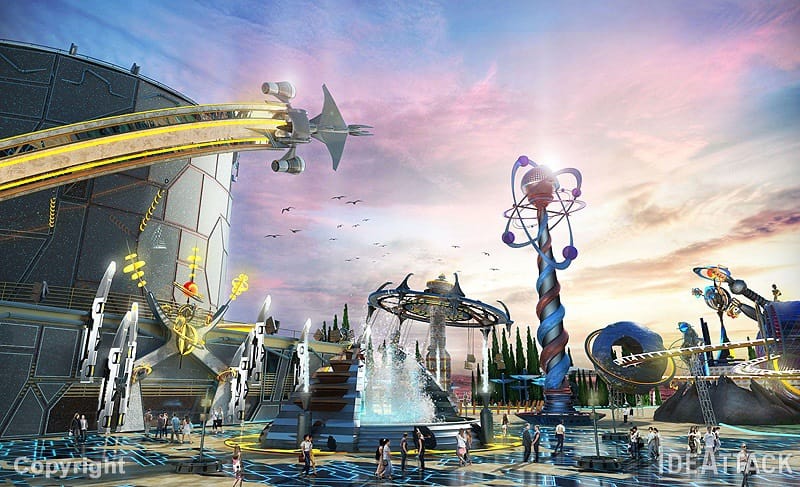The image is a highly detailed, AI-generated illustration of a futuristic amusement park, bordered by a stunning sunset with hues of reddish-pink, blue, and orange. Central to the image is a towering silver pillar, reminiscent of a 'Jimmy Neutron' structure, adorned with spiraling blue, green, and red patterns and crowned by a large red ball, giving it an atom-like design. To the left, a rocket ship, seemingly attached to a structure, trails a vivid burst of yellow flames. This fantastical park features a variety of innovative rides including a trackless roller coaster soaring through the air and a notable swing-style ride. There’s also a prominent water-themed attraction with a large spinning element and cascading water. In the foreground, miniature figures of people illustrate the grand scale of the park as they wander across what appears to be a glittering marble surface, adding to the park's otherworldly atmosphere. The bottom left corner of the image includes a visible copyright mark and the text "Idea Attack." The entire scene merges cutting-edge amusement park concepts with the captivating beauty of a dusk sky.